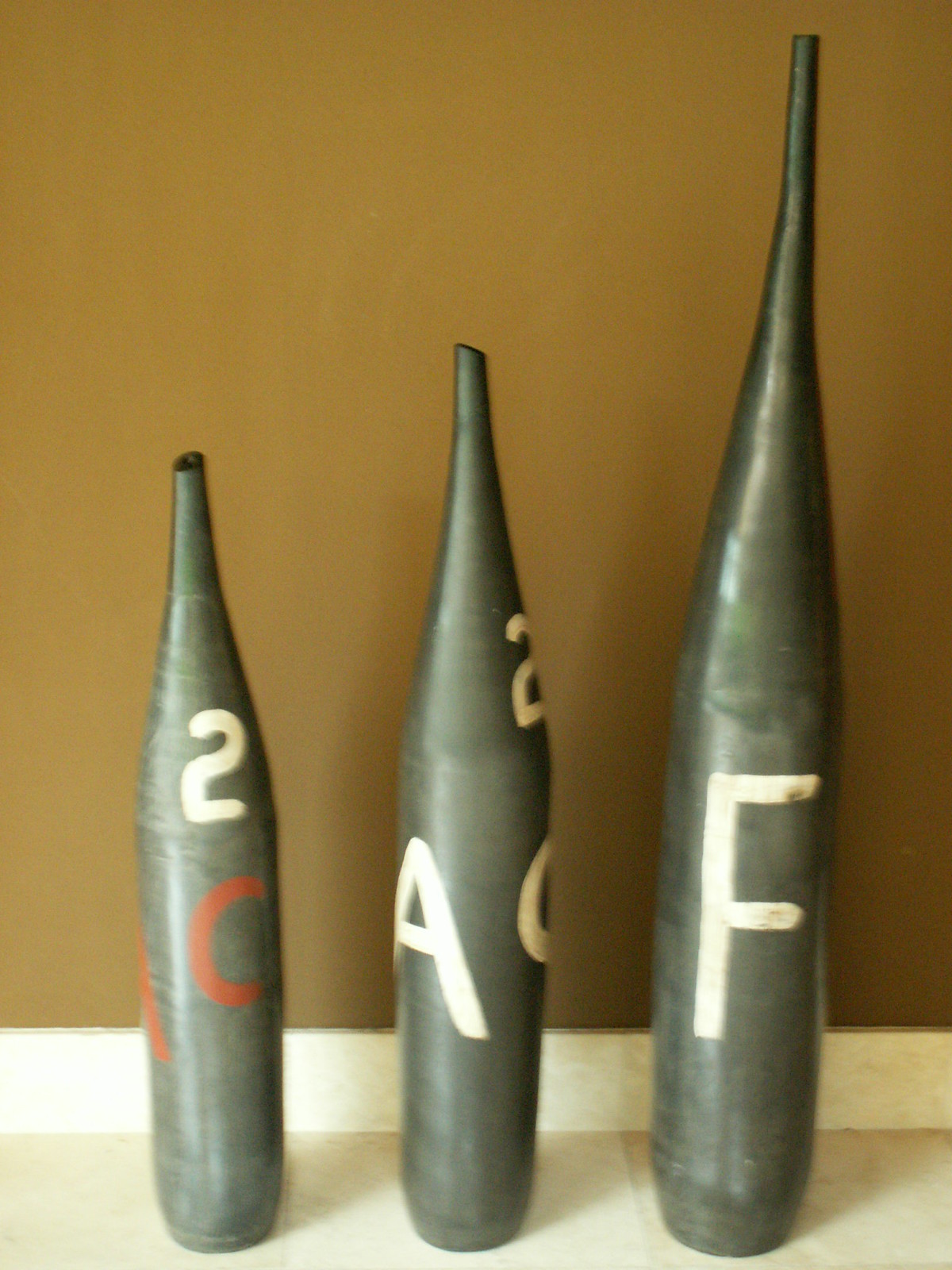The photograph features three bottle-shaped objects of varying sizes placed on a tile floor against a tan-colored wall with a white baseboard. The objects are arranged in increasing size from left to right. Each bottle is a khaki green color and cylindrical, with narrow necks that become progressively longer with each size. The smallest bottle has a white number '2' and a red letter 'C' painted on it, with another indistinguishable red letter. The medium-sized bottle displays a white number '2' and a white letter 'A,' along with another partially visible letter. The largest bottle features a white letter 'F' on its slender, elongated neck. All three have small openings at the top of their narrow necks.